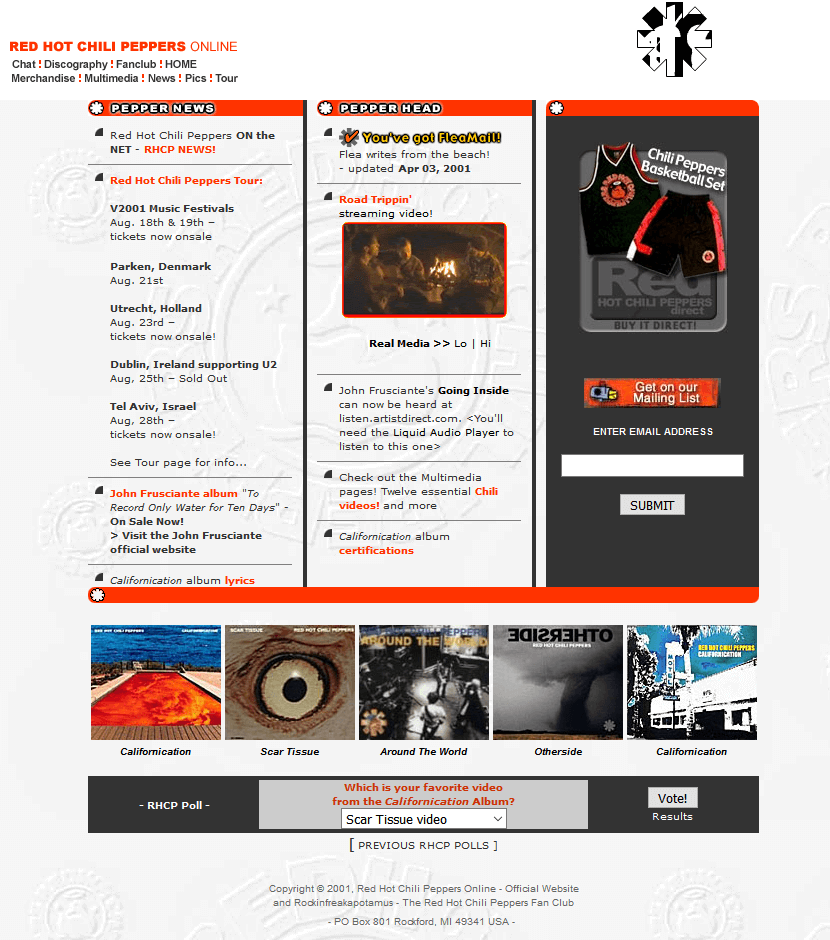**Detailed Description:**

You are on the official Red Hot Chili Peppers website, immediately greeted by the distinctive Red Hot Chili Peppers logo prominently displayed at the top. This iconic emblem resembles a stop sign with its eight pronged-edge design, and it is adorned with the band's name in striking red text.

Beneath the banner reading "Red Hot Chili Peppers Online," you find an easy-to-navigate menu offering diverse sections like Chat, Discography, Fan Club, Home, Merchandise, Multimedia, News, Photos, and Tour Dates. Each section is designed to immerse you deeply into the world of the Red Hot Chili Peppers.

The page's background features a subtle gray tone, with various instances of the Red Hot Chili Peppers logo faintly appearing throughout, providing an engaging visual theme. In the center, a section titled "Pepper News" presents the latest updates and information about the band. Here, upcoming tour dates are listed, with performances scheduled in Denmark, Holland, Dublin (Ireland), Tel Aviv, and at the V2001 Music Festival.

One link directs you to purchase John Frusciante's album "To Record Only Water for Ten Days" and provides access to his official website. In another segment, bassist Flea shares personal letters under the title "Flea Mail," forming a unique connection with the fans.

The page also features multimedia content, including the "Road Trippin'" music video available in both low and high resolutions. Additionally, you can stream John Frusciante's track "Going Inside" from ListenArtistDirect.com, though you will need the Liquid Audio Player for this feature. The multimedia section also showcases various certifications earned by their "Californication" album.

To the right, there's a promotional ad for a Red Hot Chili Peppers basketball set, featuring a sleeveless top and matching basketball shorts. Visitors can enter their email to join the mailing list and stay updated with the latest news and exclusive offers.

At the bottom of the page, five Red Hot Chili Peppers album covers serve as virtual bookmarks. These include:
- "Californication" (depicting a serene pool scene)
- "Scar Tissue" (featuring a close-up of an eye)
- "Around the World" (presented in a striking black and white design)
- "Otherside" (illustrating a tornado in a stormy black and white setting)
- Another Californication-themed cover with a blue and white background

This comprehensive overview captures the essence of the Red Hot Chili Peppers' online presence, offering fans extensive news, media, and merchandise options in a visually engaging manner.